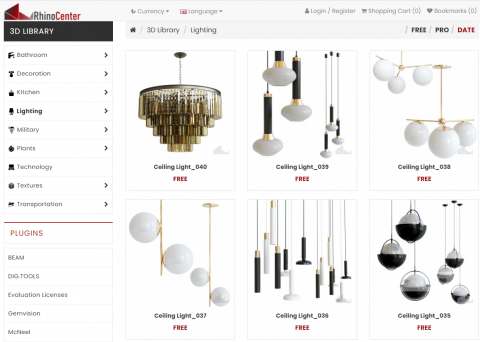The image depicts a white webpage from a catalog or online store, titled "Rhino Center" in the upper-left corner. Below this title, "3D Library" is marked, with several categories listed, including bathroom, decoration, kitchen, lighting, military, plants, and more. The "lighting" category is highlighted. To the right, there are six images of various ceiling light fixtures arranged in two rows of three. These modern and futuristic lights include designs such as chandeliers made of gold metal, hanging globe-like lamps, and slim lights. Many globes and bulbs are white, adorned with metal accents in black or other finishes. Descriptions note that some of these lights are labeled as free, with specific product codes such as ceiling light 040 in the first position and ceiling light 039 next to it. All lights hang from either long strands of wire, rods, or single brackets, showcasing varied yet cohesive elegant styles.